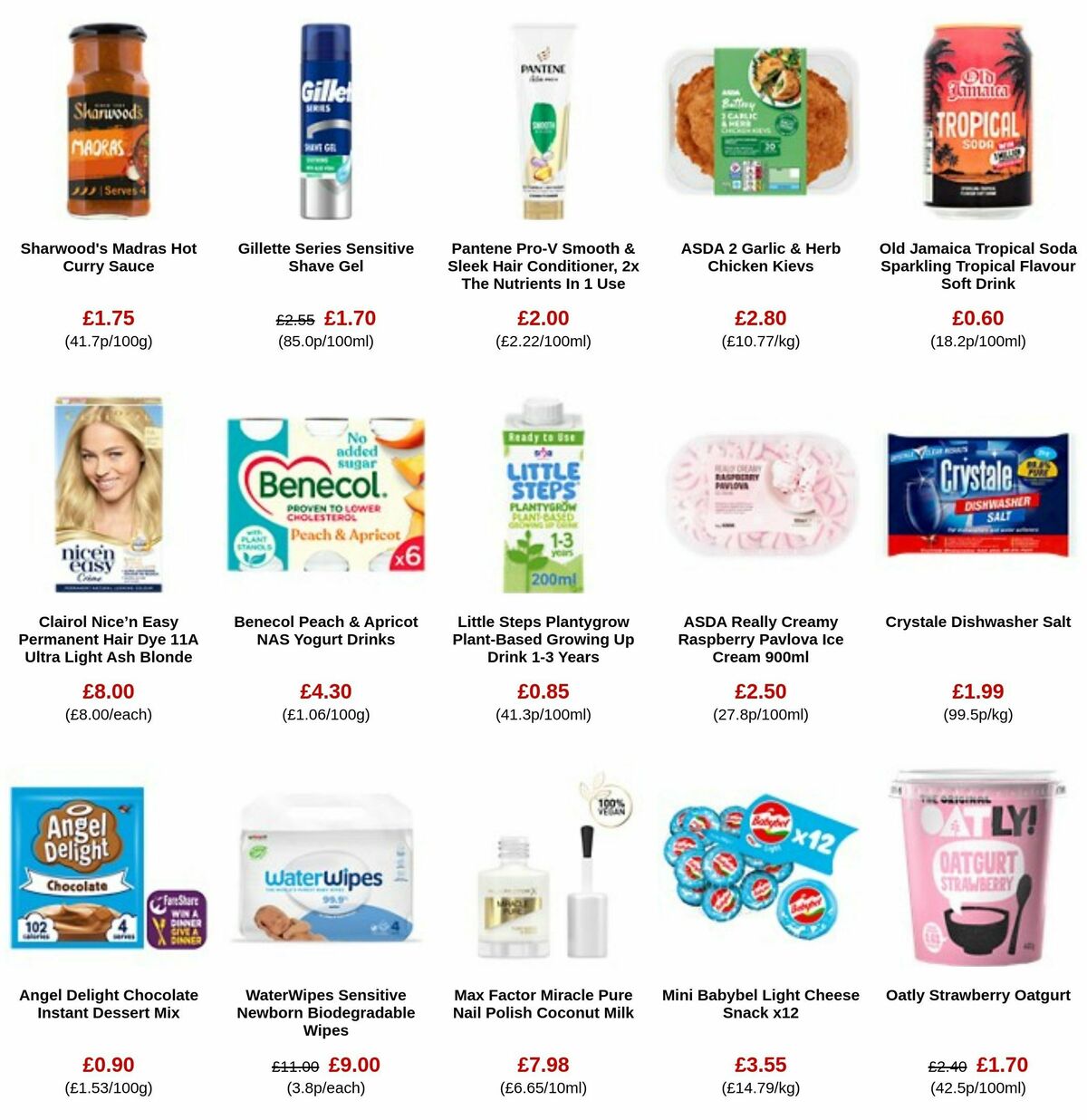The screenshot displays a webpage featuring a grid of fifteen products organized in three rows, with five products in each row. Each product is depicted with an image on a transparent background, followed by its name and price, along with either the price per 100 grams or its net weight.

- **Top Row, Left to Right:**
  1. "Shorewood's Madra's Hot Curry Sauce" priced at £1.75.
  2. "Gillette's Serious Sensitive Shave Gel".
  3. "Pantene Pro-V Smooth and Sleek Hair Conditioner".
  4. "Asda 2 Garlic and Herb Chicken Kievs".
  5. "Old Jamaica Tropical Soda Sparkling Tropical Flavor Soft Drink".

- **Middle Row, Left to Right:**
  1. (Not mentioned in the provided text).
  2. (Not mentioned in the provided text).
  3. "Nice N Easy Permanent Hair Dye, shade 11A Ultra Light Ash Blonde".
  4. (Not mentioned in the provided text).
  5. (Not mentioned in the provided text).

- **Bottom Row, Left to Right:**
  1. (Not mentioned in the provided text).
  2. (Not mentioned in the provided text).
  3. (Not mentioned in the provided text).
  4. (Not mentioned in the provided text).
  5. (Not mentioned in the provided text).

Each item listing includes an image, product name, and price. The detailed arrangement helps users easily compare products and make informed decisions.